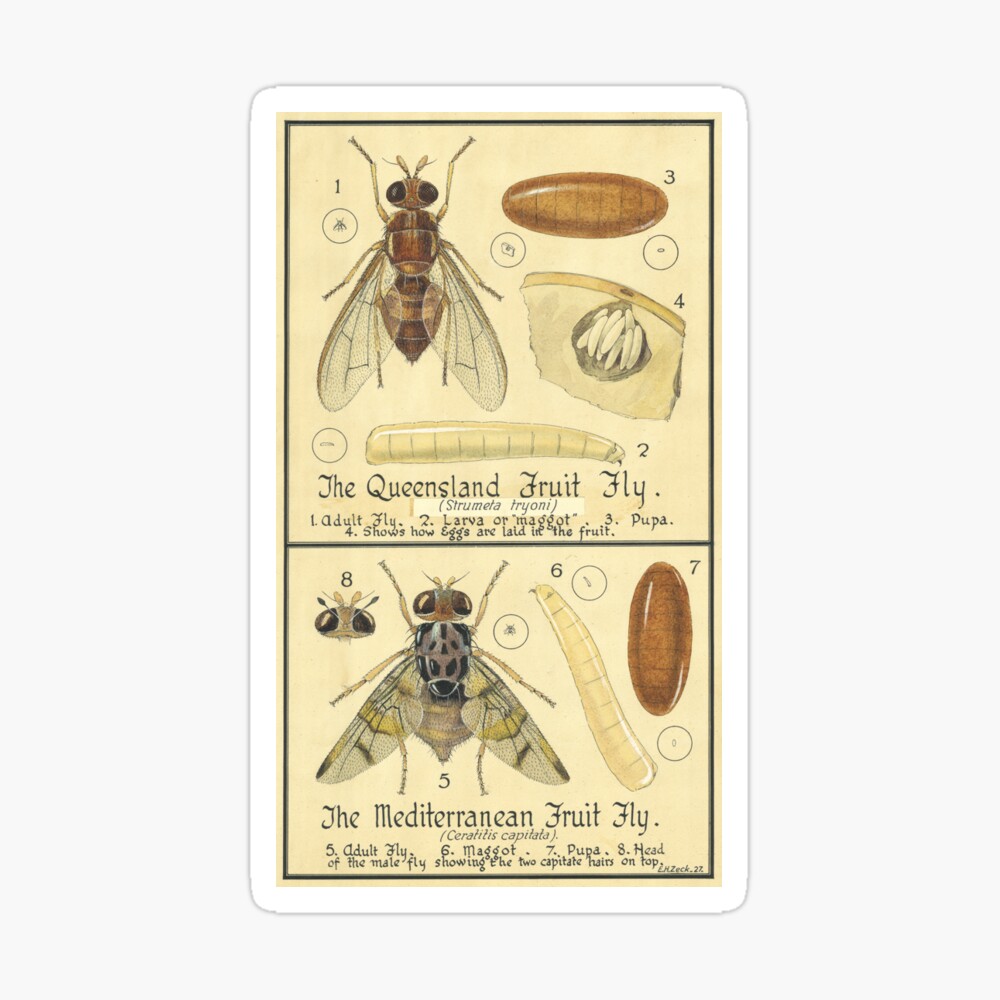The image depicts an aged manuscript, bordered in white, tan, and black, meticulously illustrating the life cycles of two fruit fly species: the Queensland fruit fly and the Mediterranean fruit fly. The top half of the manuscript, labeled with a "1," focuses on the Queensland fruit fly, detailing its life stages from egg to adult. Accompanying labels identify various stages: the white, cylindrical larvae or maggots; the brown pupae with black stripes; and an image depicting eggs laid in decomposing fruit. The adult Queensland fruit fly is light brown in color. 

The bottom half of the manuscript, divided by a number "8," describes the Mediterranean fruit fly. It features a head illustration of the male fly with prominent eyes and antennae. This section also showcases the fly’s stages: the maggot stage, the brown pupae, and the detailed anatomical depiction of the fly's head. The adult Mediterranean fruit fly possesses a body with a black and sickly yellow color, resembling a cross between a Vader mask and a Spider-Man mask due to its green and yellow wing patterns. A legend at the bottom clarifies the stages and elements displayed, providing a comprehensive overview of both species' developmental stages.